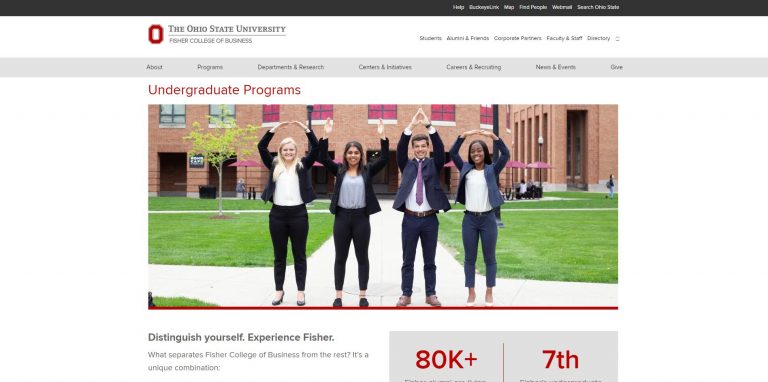This image is an advertisement for the Ohio State University's Fisher College of Business. The foreground features a diverse group of four students—two white females, one Hispanic female, and one Black male—enthusiastically forming the letters "O-H-I-O" with their arms, mimicking the iconic YMCA pose. Behind them, a verdant university lawn can be seen, adorned with picnic tables where students are engaged in conversations and activities. One of the stately campus buildings stands in the background, lending an academic atmosphere to the scene.

At the bottom of the image, there are some textual elements that highlight various facets of Fisher College. The caption reads, "Distinguish yourself. Experience Fisher. What separates Fisher College of Business from the rest? It's a unique combination." Additionally, there are metrics including "80,000+" and another snippet indicating a "seventh" place ranking, although the specific context for these numbers is partially obscured. The visual and textual elements collectively emphasize the college's commitment to diversity, comprehensive academic programs, and distinguished status in business education.